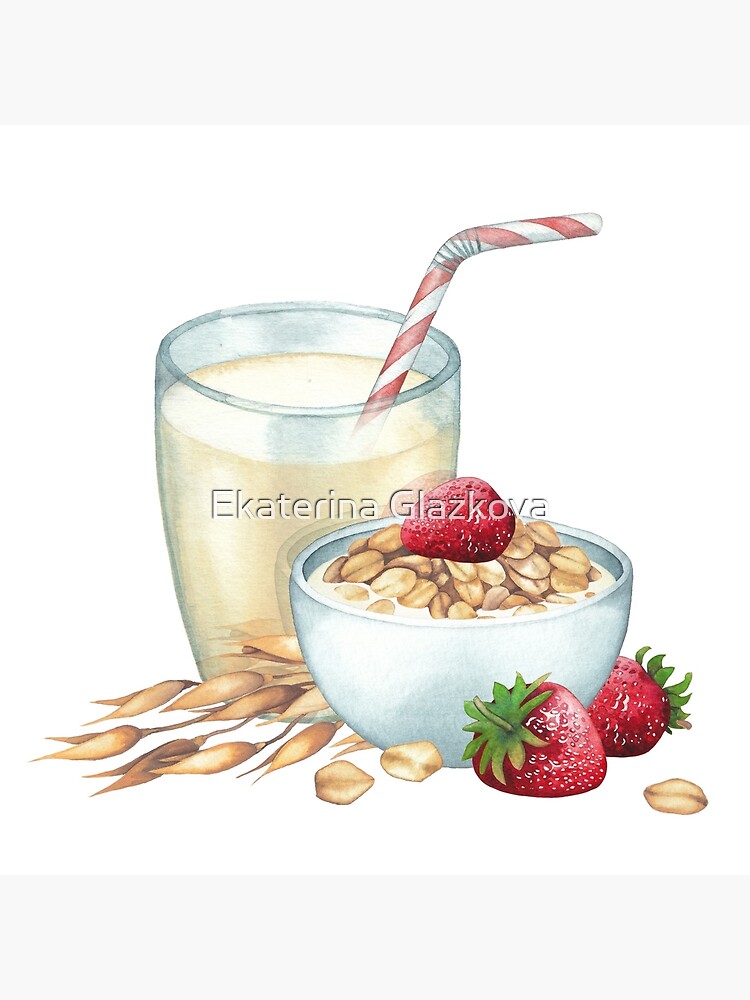This artistic image, likely a colored pencil drawing by Ekaterina Glazkova, features a meticulously detailed still life. At the center is a clear cup filled with light brown liquid, distinguished by a red-and-white striped bendable straw protruding to the right. Adjacent to the cup is a white or gray bowl containing what appears to be natural cereal or oats, topped with one vibrant red strawberry. Surrounding the bowl are additional strawberries—two positioned on the bottom right, each showing off their green tops and seeds depicted with white dots. Scattered near the bowl are loose grains or flakes, with a prominent brown wheat stalk sitting between the bowl and the glass. The background is kept plain white, emphasizing the delicate interplay of color and texture within the composition.